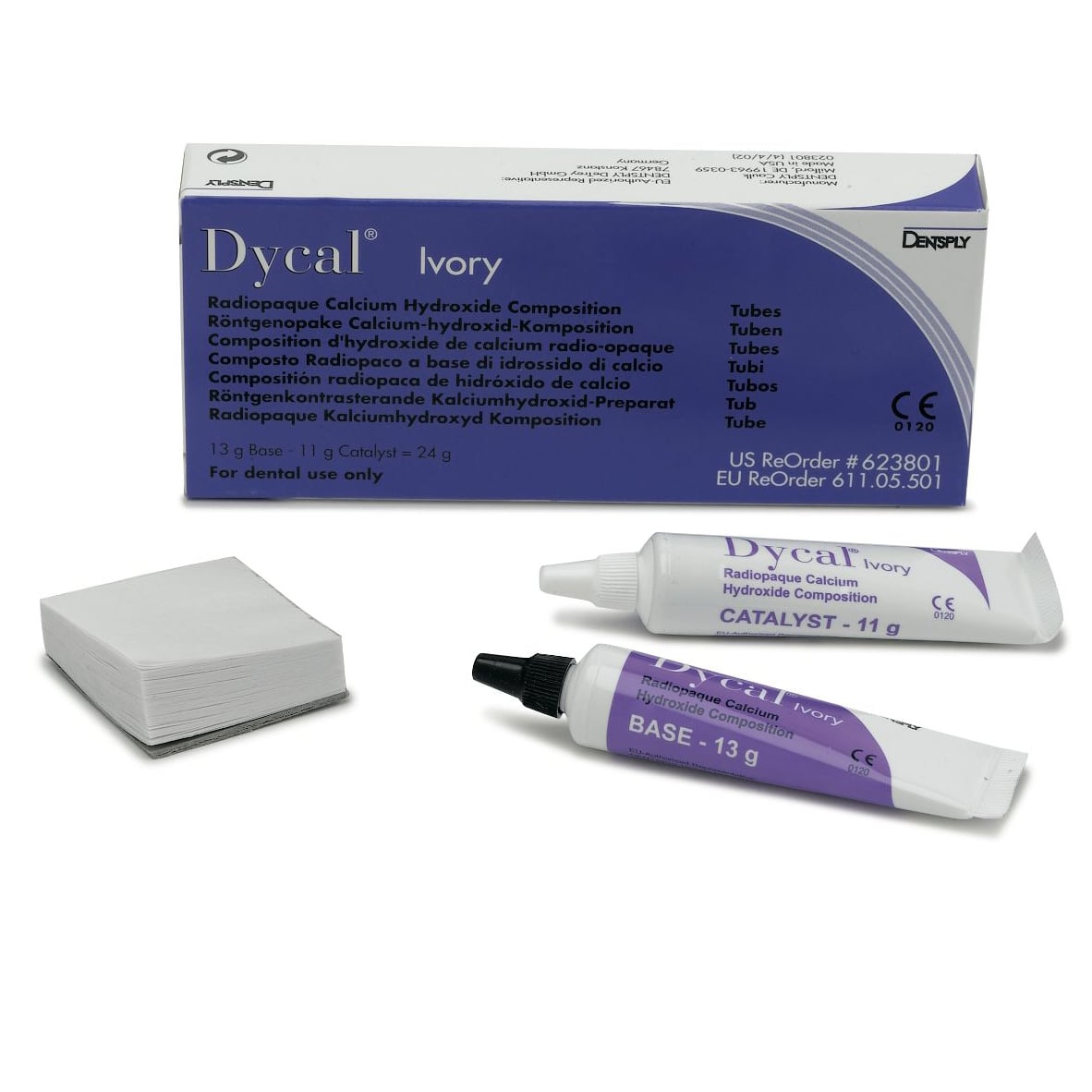The image depicts a dental product set against a plain white background, likely arranged for advertisement purposes. The main feature is a rectangular, navy blue, and white box labeled "DICAL" in large text, with "Ivory" below it. The box prominently displays "Radiopaque Calcium Hydroxide Composition" alongside text that appears in multiple languages, indicating its chemical composition and usage. Additional details on the box include "13-gram base" and "11-gram catalyst," which add up to "24 grams," with a clear indication that the product is "for dental use only." U.S. reorder number 623801 and an EU reorder number 611.05.501 are also visible.

Accompanying the box are two tubes and a white pad that resembles gauze or cotton wipes. The tubes are similarly labeled "DICAL Ivory Radiopaque Calcium Hydroxide Composition." The white tube with purple print is marked "Catalyst 11-gram" and has a white cap, while the white tube with a purple band and black cap is labeled "Base 13-gram." These tubes are likely intended for use together in a dental procedure. The white pad, although less clearly defined, appears to be an accessory for the application or cleanup process associated with the dental product.